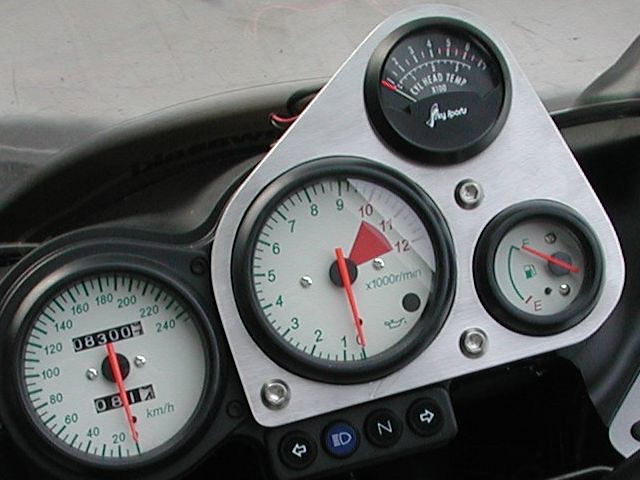The photograph captures the top view of a meticulously designed device, showcasing a blend of silver and black hues, highlighted under a well-lit setting. The device features several notable elements: prominently, there are four round dials. 

On the left, a large dial displays measurements from 0 to 240 with a red needle currently pointing at 83,007 and 0814 kilometers at its base. Adjacent to it, the center dial is marked from 1 to 12, also including a red needle, where the numbers 10 to 12 are distinctly highlighted in red, indicating a critical range. Above this, the topmost dial ranges from 1 to 10, labeled "CTE Head Temperature," providing precise temperature readings.

Lastly, the bottom right corner houses the smallest dial which measures fuel levels, ranging from 'Full' to 'Empty.' Complementing this sophisticated array are some black, soft-touch buttons situated towards the bottom of the device, adding to its functional design.